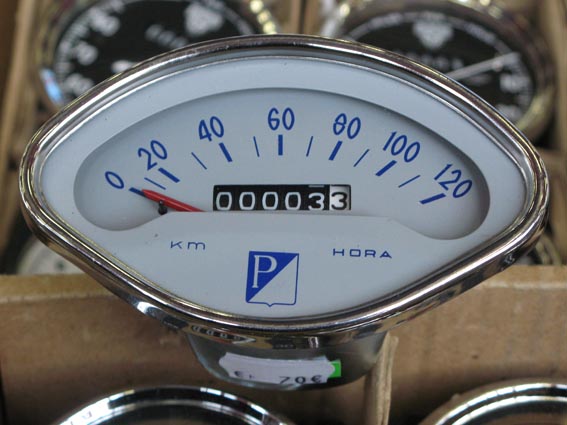The image showcases a close-up of a speedometer with a white face, encased in a steel outline. The speedometer measures speed in kilometers per hour (km/h), with markings at intervals of 0, 20, 40, 60, 80, 100, and 120 km/h. There is a prominent red needle pointing to zero. The device features blue numerals against the white background, providing clear readability. The speedometer includes the text "km/h" in white along with a "P" logo positioned at the top left corner. The background of the shot appears to be a plain white surface, possibly outlining the steel casing.

The bottom of the image reveals parts of the packaging, including cardboard boxes and other components, suggesting that the speedometer is part of a kit typically used in custom motorbike builds. Additionally, there are two other steel-cased speedometers visible at the top, hinting at possibly different variants or additional instruments. The overall setup displays the product in a neat, organized manner, emphasizing the details and quality of the speedometer.